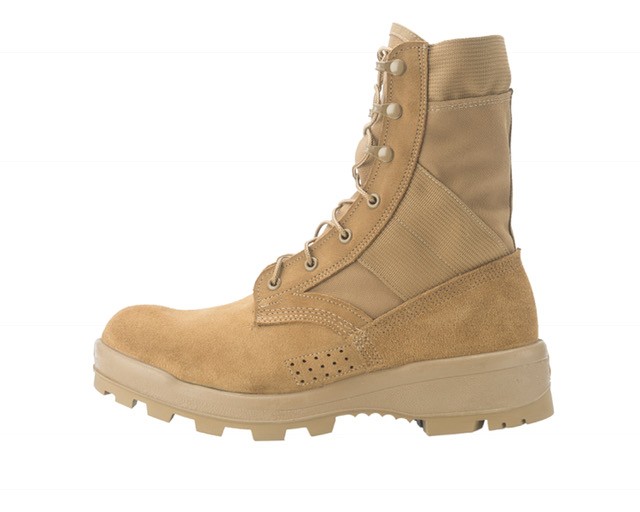The image is a high-quality, color photograph of a single tan combat boot, positioned in the center against a white background, effectively showcasing its details. The boot, reminiscent of military footwear such as those used in desert environments, features a thick tan lug sole and a combination of suede and possibly Gore-Tex or nylon materials. The suede encompasses the toe, heel, and the placket that includes eyelets and brass hooks. There are four grommets followed by three hooks for the laces, which extend up to mid-calf, ensuring a secure fit. The upper part of the boot also has breathable perforations, about fifteen tiny holes, for aeration situated near the arch. The back of the boot appears to be made of a stretchy nylon or canvas material, enhancing comfort and flexibility. This boot's rugged sole suggests suitability for outdoor work, while the materials hint at weather-resistant and durable construction.